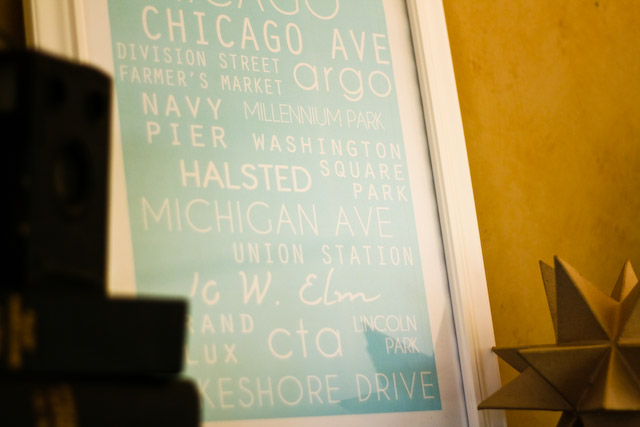The photograph captures a detailed interior setting. Dominating the scene is a white-framed artwork leaning against an orange-gold wall. The framed piece features a light blue background with a list of various locations in Chicago written in white text, including Chicago Avenue, Division Street, Farmers Market, Navy Pier, Millennium Park, Washington Square Park, Halsted, Michigan Avenue, Union Station, and Lincoln Park. On the lower right corner of the frame, there is a distinctive gold star with several sharp points. Additionally, on the left side of the frame, there is a dark, blurry object that partially obscures the view of the sign. The overall composition suggests a carefully curated display, possibly on a shelf or mantle, with attention drawn to the Chicago-themed artwork.